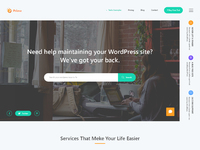The image is a small, blurry screenshot of a website, making the details difficult to discern. The visible elements include a prominent line of text reading, "Need help maintaining your WordPress site? We've got your back." This text is situated above a search field, which features a gray button next to it. The background image shows the back of a middle-aged woman with a denim button-up shirt, appearing to type on a laptop in front of a window. Below the search field is a white bar with the text, "Services that make your life easier," where the word "make" is underlined with a green dash. The rest of the webpage includes small, illegible text, various menu options at the top, and multicolored circular icons scattered across the page. The overall impression is that of a cluttered and unfocused website snippet, roughly the size of a postage stamp.